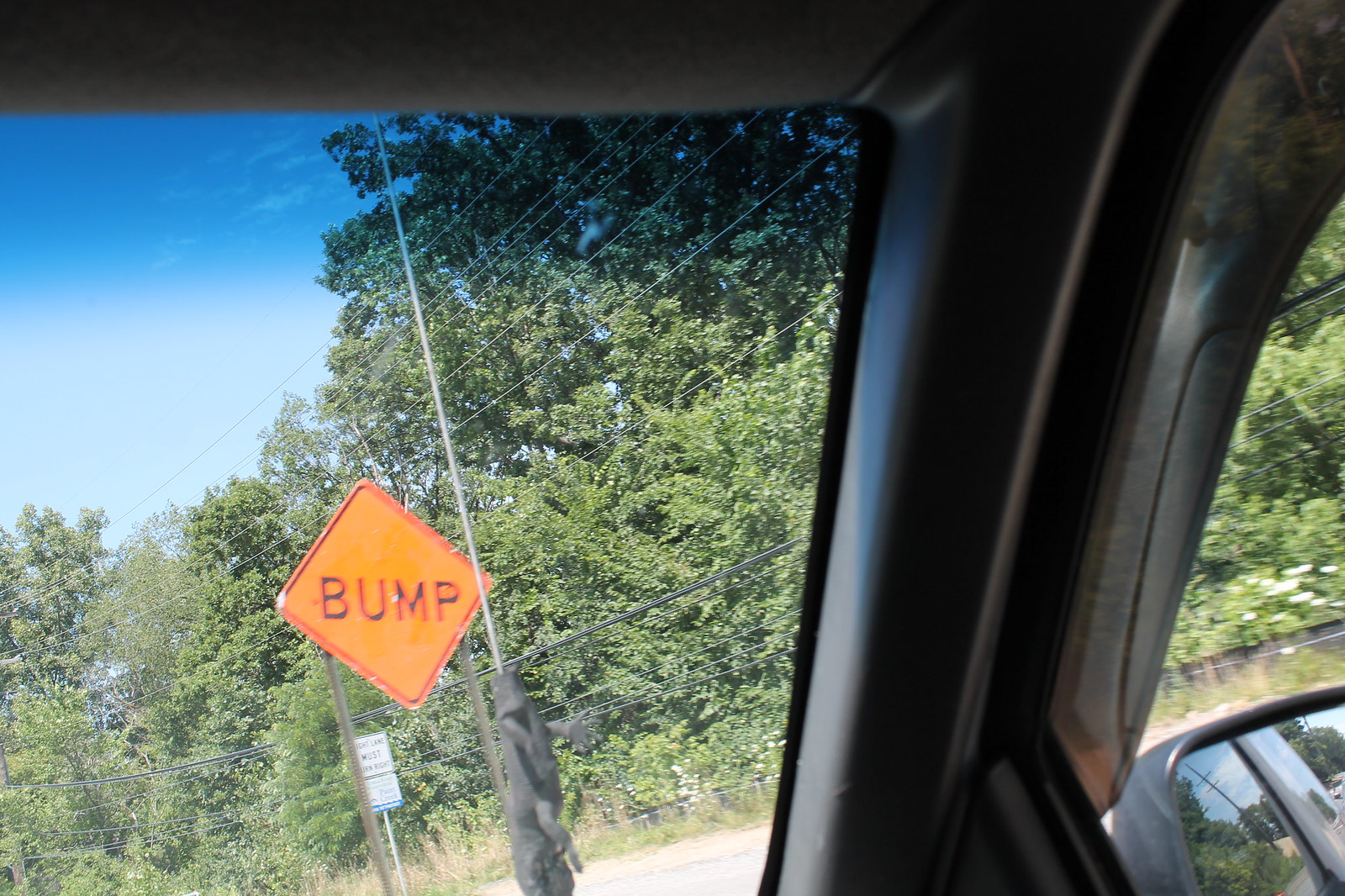The image captures a view from inside the passenger side of an American car, looking through the front windshield and right window. Dominating the scene is a diamond-shaped, orange sign with black text that reads "Bump," located just outside the windshield on the right. Beneath it, a smaller, rectangular white sign with green text and a blue strip at the bottom, possibly containing parking information, is visible but too small to decipher. A thin pole with black fabric at its base, potentially a discarded sweatshirt, stands closer to the vehicle. The background is lush with overgrown greenery and tall trees, accompanied by wooden poles that support numerous power lines crisscrossing the scene. The sky is mostly clear with a few scattered clouds, creating a bright and sunny atmosphere. The car’s rearview mirror on the right window reflects the street behind, showing another wooden power pole and more trees. The photo, taken from the perspective of someone seated inside the car, provides a detailed snapshot of a serene yet tangled roadside environment.